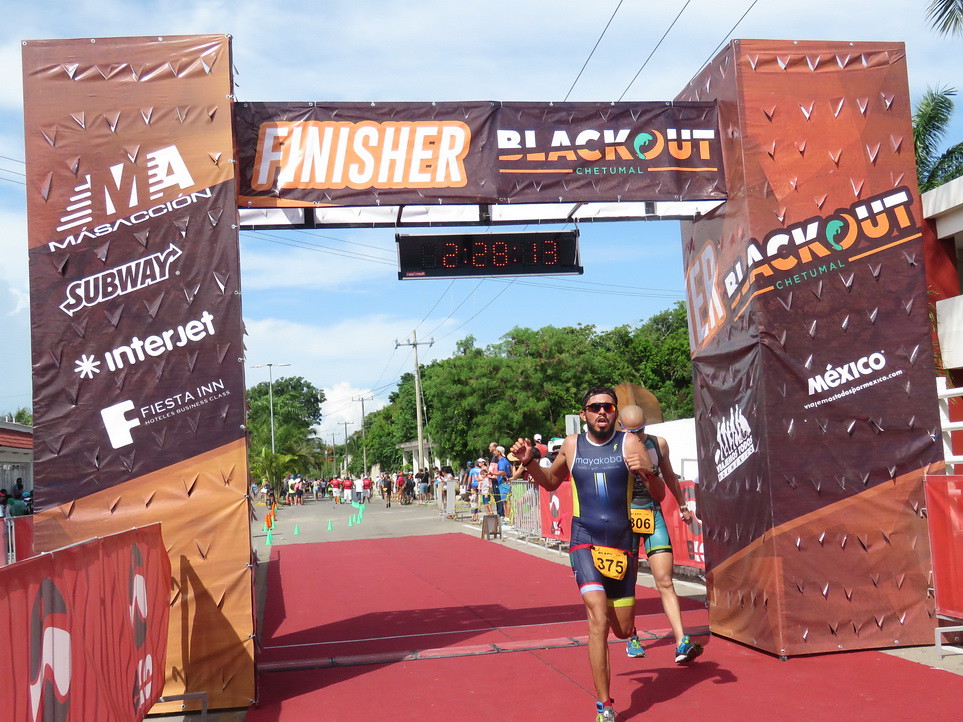This detailed photograph captures the climactic moment of a race, as runners cross the finish line under a broad, towering archway. The archway, constructed from two large, box-like barriers on either side, is primarily red, brown, and light brown, rising to a height of approximately 12 to 15 feet. This forms a dramatic frame for the runners, with the horizontal connecting bar emblazoned with the word "FINISHER" and the word "BLACKOUT" prominently positioned above the clock that displays the finishing time of 2:28:13. Advertisements for Subway, Interjet, Fiesta Inn, and Mexico are visible on the barriers.

At the bottom center of the image, the main focus is a man with light brown skin, sporting sunglasses, black hair, a mustache, and a beard. He is dressed in a dark navy tank top with "Mayakoba" printed on it and matching running shorts. A sign with a gold background and the number 375 is affixed around his hips, indicating his participation number. The pathway beneath him features a distinctive red mat, contrasting with the standard road surface visible further into the background.

Immediately behind this prominent runner, slightly to the right, is a bald man of Caucasian descent, wearing a blue jersey and shorts, marked with the number 806. The scene extends to include more runners approaching the finish line and a crowd of spectators, some standing on the sidelines and others watching intently. Green trees and lampposts frame the sides of the road, and a clear blue sky stretches overhead, underscoring the daytime setting of this outdoor event.